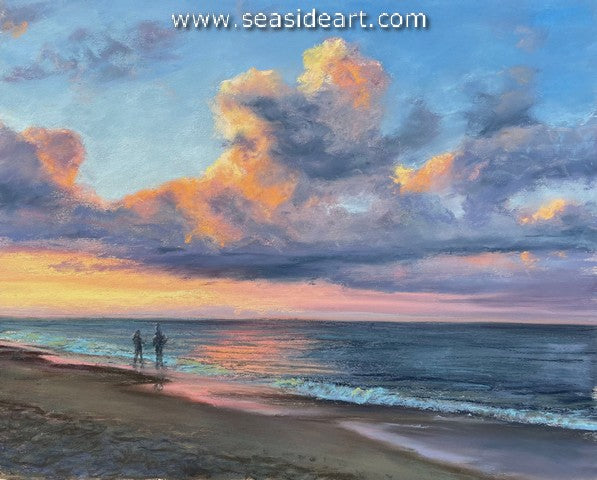The detailed painting showcased in this advertisement for the artist's website, www.seasideart.com, features a thunderous and dramatic evening sky. At the very top, written in lowercase white-ish letters, the website address is prominently displayed. Swirling clouds in hues of dark blues, grays, light blue, and gold dominate the heavens, with the horizon bathed in a sunset's glow. To the left, vibrant shades of gold and yellow peek through turning to purple as the scene extends to the right. The ocean mirrors these stunning colors, reflecting the sky's drama on its mildly rippling surface near the shoreline. 

In the distance, the silhouette of two people walking along the very edge of the water can be seen, with tiny waves gently lapping at their feet. The sandy foreground, dotted with footprints and shells, appears darker, highlighted by the approaching dusk. The perspective suggests a wide and encompassing view of the serene yet powerful seascape, marked by the interplay of light and shadow as day transitions into night.